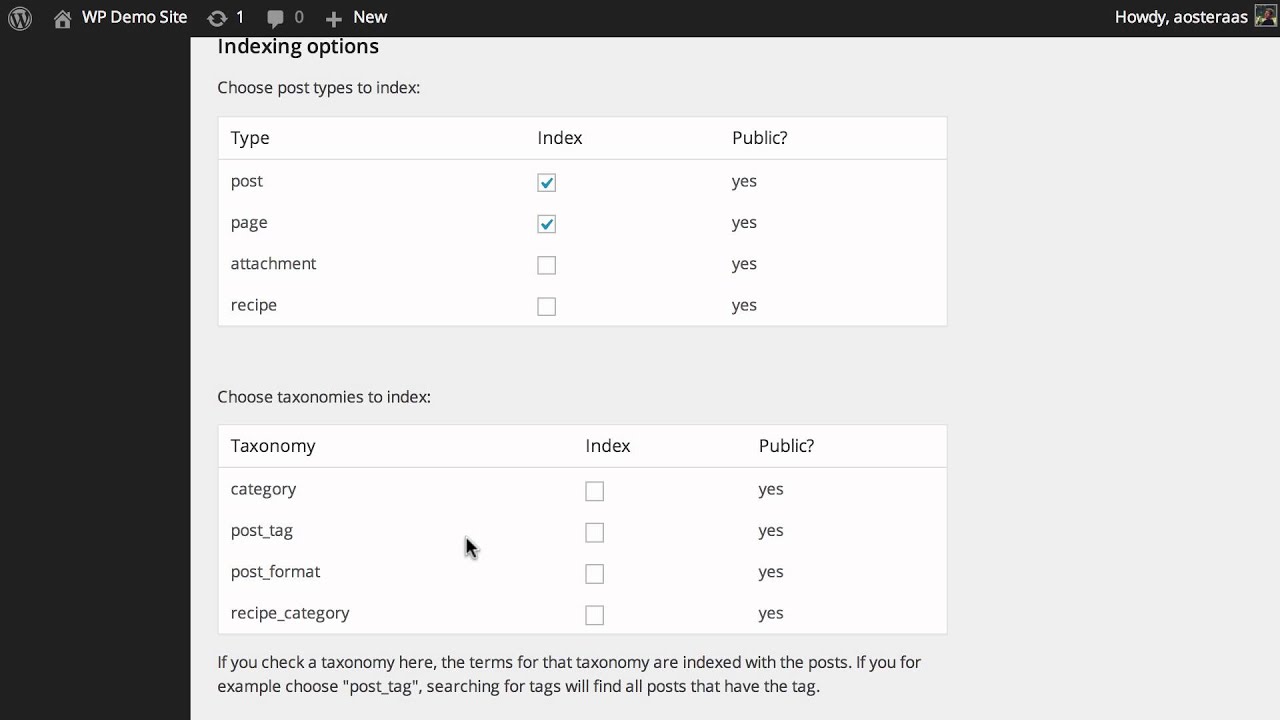The webpage features a detailed indexing option menu set against a contrasting black background. The top segment of the page maintains a sleek black strip, accompanied by a left-aligned black column extending vertically from top to bottom and measuring approximately an inch and a half in width.

In the upper left corner sits a white circle containing a bold black "W." Adjacent to this circle is a white house icon followed by the label "WP Demo Site." Further to the right, a gray circle with a white number "1" is observed, followed by a gray chat box icon labeled with a gray "0." Continuing in this sequence is a gray plus symbol beside the word "New."

On the far left side, there is a greeting in white text: "Howdy, OASTERAAAS," accompanied by an icon depicting a person's image. 

The pop-up menu occupying the top left corner presents the title "Indexing Options" in black text, with the subsequent instruction, "Choose Post Type to Index." The layout below features three vertically-aligned columns: "Type," "Index," and "Public?" Under "Type," the options listed are "Post," "Page," "Attachment," and "Recipe." Corresponding to these entries, the column under "Index" displays checked blue boxes for "Post" and "Page," while "Attachment" and "Recipe" remain unchecked. The "Public?" column consistently reads "Yes" for all options.

Below, the section "Choose Taxonomies to Index" mirrors the format, with column headers "Taxonomy," "Index," and "Public?" Listed under "Taxonomy" are "Category," "Post_Tag," "Post_Format," and "Recipe_Category." The "Index" column here contains four unchecked white boxes, and the "Public?" column features "Yes" for each taxonomy option.

A note beneath clarifies: "If you check a taxonomy here, the terms for that taxonomy are indexed with the posts. If you, for example, choose (Post_Tag), searching for Tags will find all posts that have the tag."